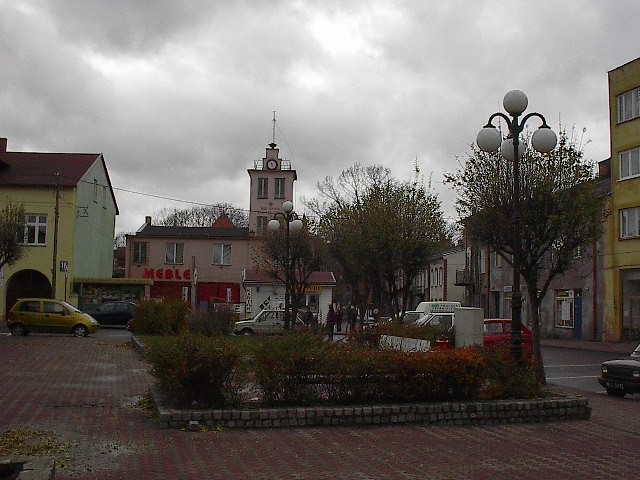The photograph depicts a charming small-town downtown area, with an old-world European ambiance. The focal point of the scene is a brick-paved central square surrounded by historic buildings, suggesting a communal gathering spot likely more vibrant on sunnier days. The environment appears quiet and deserted with only a few parked cars, likely a reflection of the stormy, overcast weather, as the gray sky hints at impending rain.

Flanking the square are buildings over a century old, painted in a variety of colors—gray stone and a notable yellow façade catching the eye. Among these is a distinctive pink building featuring an old steeple-cum-clock tower, possibly a repurposed schoolhouse or church. Stone-edged planters with bushes and trees add greenery to the brick walkway, and several ornate street lamps, with multiple spherical lights, add a historic touch to the scene. The word "Meeble" in red stands out on one of the buildings, complemented by red garage doors beneath a tower section.

Despite the potential for activity, particularly in better weather, the current scene emphasizes a tranquil, almost abandoned quality, making the viewer feel as if they have stepped into a nostalgic moment within this quaint European town.